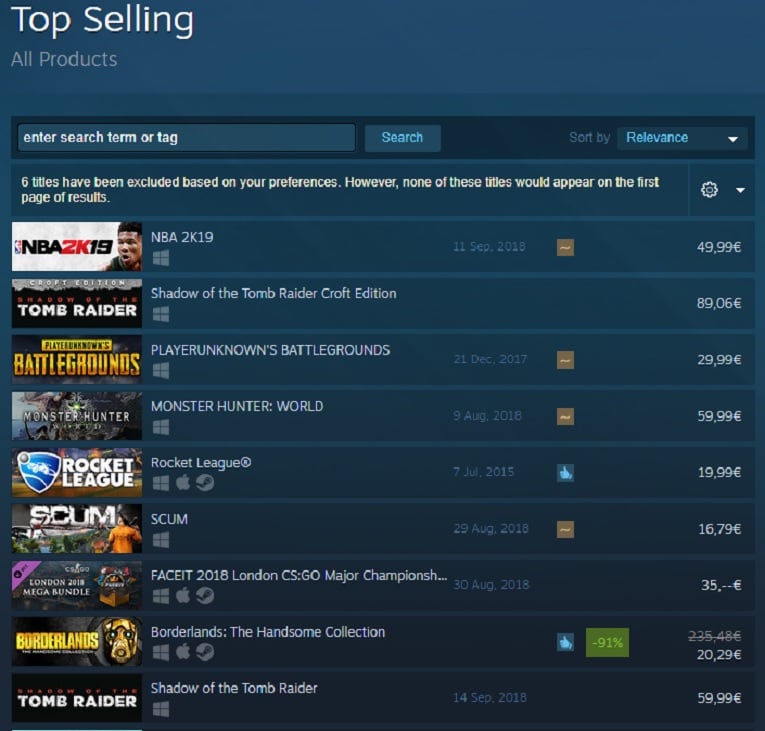A screen capture from a website displaying top-selling product listings. The page features a mid-toned navy background with various shades of blue and white highlight elements. At the top of the page, in white font, "Top Selling" is displayed next to an "All Products" option. Below this, there's a search bar with a placeholder text in white, prompting users to "enter search term or tag," accompanied by a blue search button. Next to it, there's another blue box labeled "Sort by relevance" with a white dropdown arrow, followed by another blue box stating, "Six titles have been excluded based on your preferences; however, none of these titles would appear on the first page of results," accompanied by a white cogwheel icon.

Scrolling down, the page showcases various sporting events and video game titles alongside images and prices. Key listings include:

1. **NBA 2K19**:
   - Image of an African-American gentleman.
   - Release Date: September 11, 2018.
   - Price: £49.99 (highlighted in an orange box with a white squiggle).

2. **Shadow of the Tomb Raider: Craft Edition**:
   - Red, white, black, and silver graphics with a Microsoft Windows icon.
   - Price: £89.06.

3. **PlayerUnknown's Battlegrounds (PUBG)**:
   - Black background with gold font.
   - Release Date: December 21, 2017.
   - Price: £29.99.

4. **Monster Hunter: World**:
   - Graphic depicting a pirate ship and a skull.
   - Release Date: August 9, 2018.
   - Price: £59.99.

5. **Rocket League**:
   - Stadium background with a blue and white shield.
   - Release Date: July 7, 2015.
   - Price: £19.99 (with a blue thumbs-up icon).

6. **Scum**:
   - Black background with people dressed in orange and some plants.
   - Release Date: August 29, 2018.
   - Price: £16.79.

7. **Face It 2018 London CS:GO Major Championship**:
   - Graphic of a box with overflowing items.
   - Release Date: August 30, 2018.
   - Price: £35.

8. **Borderlands: The Handsome Collection**:
   - Gold and black background.
   - Blue thumbs-up icon and green text indicating a 91% discount.
   - Price: £20.29.

9. **Shadow of the Tomb Raider**:
   - Black, red, and white imagery.
   - Release Date: September 14, 2018.
   - Price: £59.99.

This image mostly showcases video games and a few sporting events, with key details such as dates, prices, and specific graphical elements highlighted for each product.